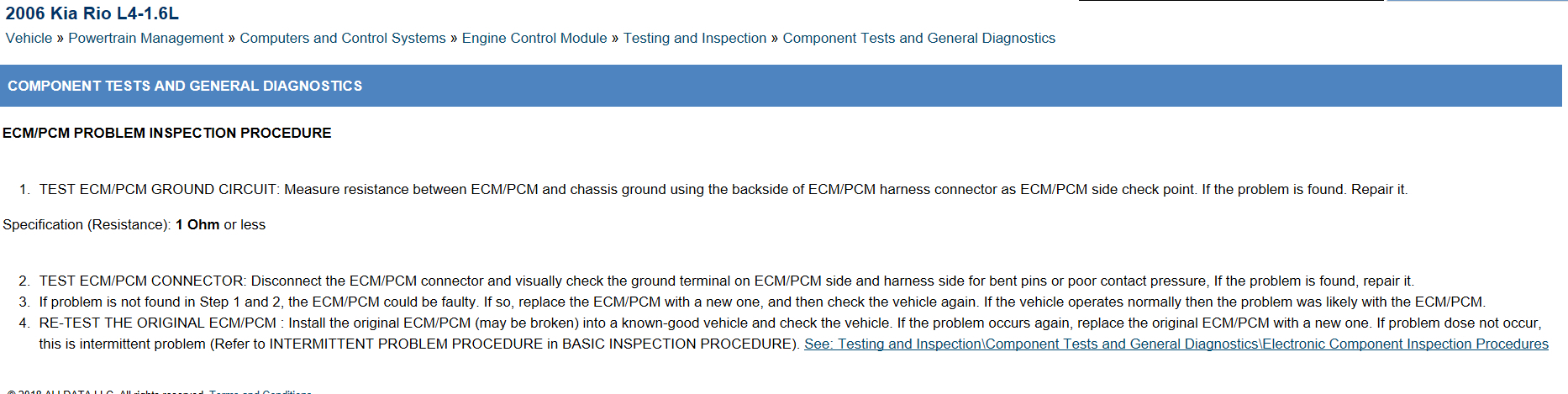A wide, rectangular image contains a predominantly white background. In the upper right-hand corner, there is a black horizontal line with a shorter gray horizontal line to its right. The upper left-hand corner of the image displays the text "2006 Kia Rio L4-1.6L" in blue font. Directly below this are the words "Vehicle > Powertrain Management > Computers and Control Systems > Engine Control Module > Testing and Inspection > Component Tests and General Diagnostics" also in blue font.

Beneath this text is a blue-shaded rectangular bar with the phrase "Component Tests and General Diagnostics" written in white font. Following this, on the white background, the heading "ECM/PCM Problem Inspection Procedure" appears in black font, subsequently followed by four bullet points in black font as well.

1. The first bullet point starts with "TEST ECM/PCM GROUND CIRCUIT:" in all caps. Below it, the instruction "Measure resistance between ECM/PCM and chassis ground using the backside of ECM/PCM harness connector as ECM/PCM side checkpoint. If the problem is found, repair it." is written in sentence case. There is a space below this instruction, followed by "Specification (Resistance): 1 ohm or less" in parentheses.

2. The second bullet point is labeled "TEST ECM/PCM CONNECTOR" in all caps, followed by additional text to the right.

3. The third bullet point starts with "If problem is not found in step one and step two, the ECM/PCM could be faulty," followed by more text.

4. The fourth bullet point, "RETEST THE ORIGINAL ECM/PCM" in all caps, is followed by more instructions. The second row of text in this bullet point ends with the words "See Testing and Inspection > Component Tests and General Diagnostics > Electronic Component Inspection Procedures" in blue font.

The image cuts off some text at the lower left-hand side.